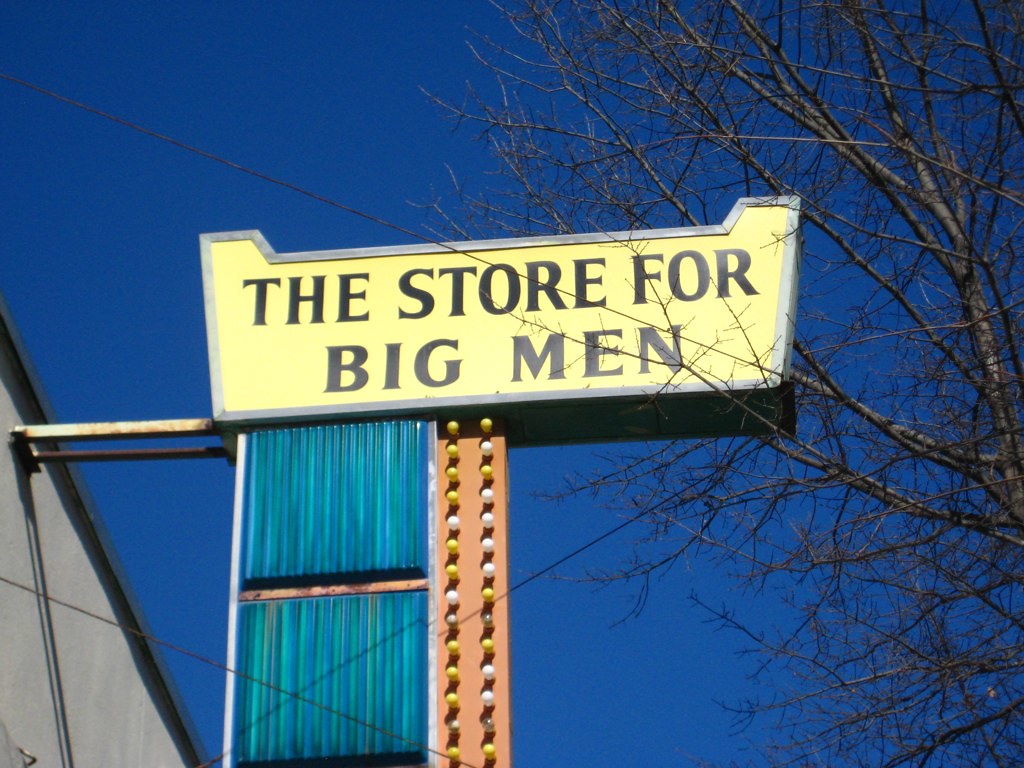This photograph captures a sign mounted on top of a building. The sign itself boasts a predominantly rectangular shape, accentuated by a sleek silver border and a bright yellow background. Bold black text reads, "The Store for Big Men," clearly announcing the store's specialty. Surrounding this text are a series of yellow and white bulbs set against an orangish backdrop, adding an eye-catching element. To the left of the sign, an array of blue squares of indeterminate purpose adds another layer of visual interest. The sign is securely fastened to the building with sturdy metal bars on its left side.

The background features a vivid deep blue sky, which contrasts strikingly with the other elements in the image. On the right side of the photograph, a leafless tree, with its intricate network of branches and twigs, is prominently visible. Additionally, a power line cuts diagonally across the picture from the upper left to the mid-right, subtly adding to the urban landscape captured in this scene.